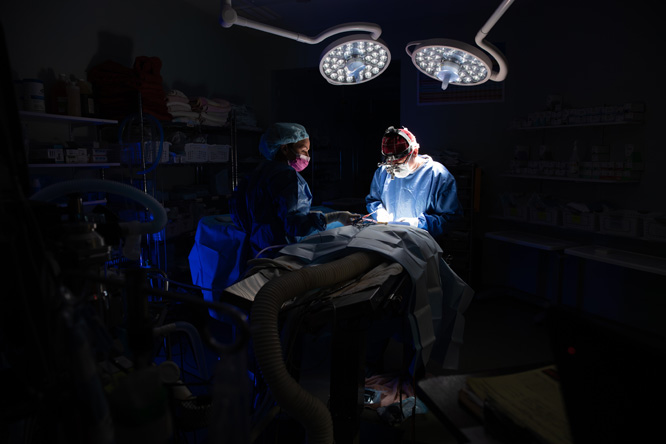In an eerily dark operating room or laboratory, illuminated only by a focused light on the central operating area, two medical professionals are meticulously working on a peculiar subject. The primary surgeon, positioned slightly to the middle-right, wears magnification glasses, a blue surgical cap tightly securing their hair, blue scrubs, white gloves, and a surgical mask, leaning intently over the subject. Beside them stands a surgical assistant, donned in a blue hairnet, pink mask, and blue scrubs. The room's periphery reveals vague outlines of machinery, shelving, and the floor, contributing to the unideal dim setting. On the gurney, what appears to be a giant earthworm or large tentacle lies under the surgical team's scrutiny, adding an enigmatic twist to the scene.